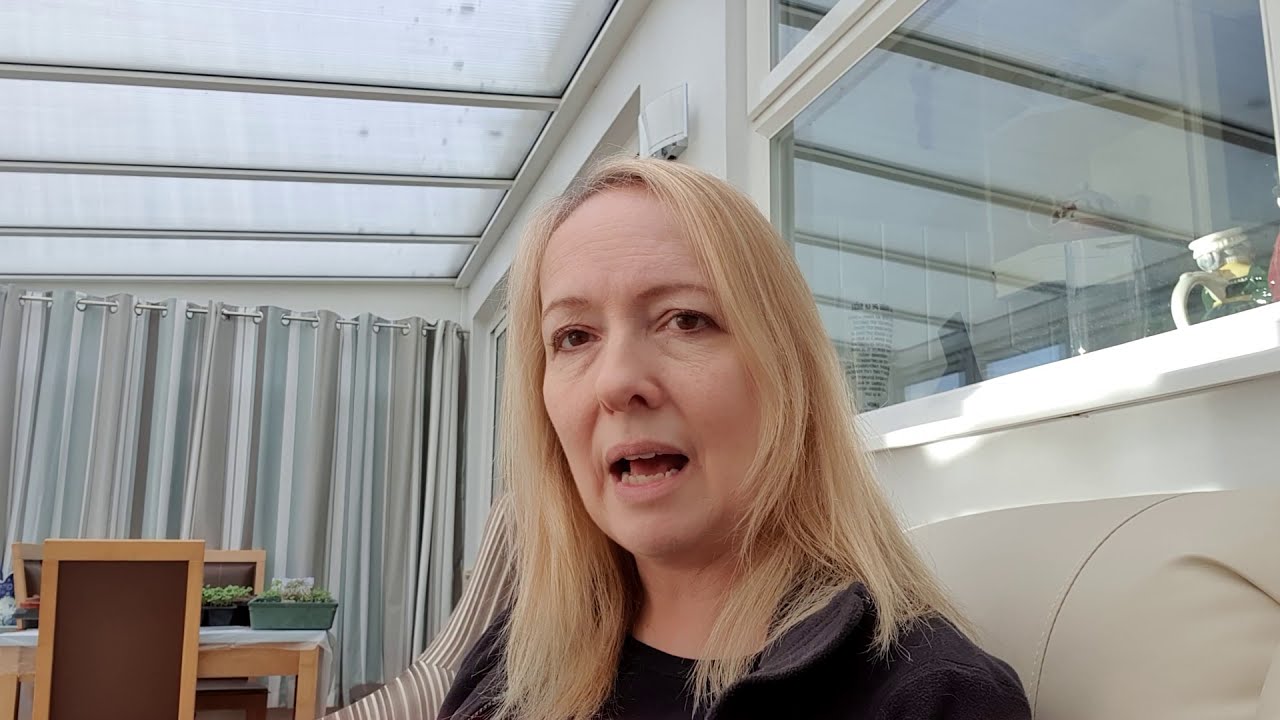The image captures a woman with blonde hair and brown eyes, sitting on a tan couch in the center of a room, positioned as if she's on a video call. She is wearing a black shirt and has a peculiar expression with her mouth open, possibly reacting to something. Behind her and to her right, there is a window with brown, green, tan, and white blinds, and a tan or yellow cup resting on the windowsill. To her left, a wooden table surrounded by wooden chairs with perhaps a bit of brown leather can be seen. The table holds various green plants in gray and black plant holders. Above the table, there are blue-gray curtains. The room possibly has a sunroof or a glass ceiling, allowing sunlight to pour in, giving a bright, airy feel to the space. Overall, the detailed setting amplifies the impression of a casual, in-the-moment snapshot within a cozy, well-lit room.